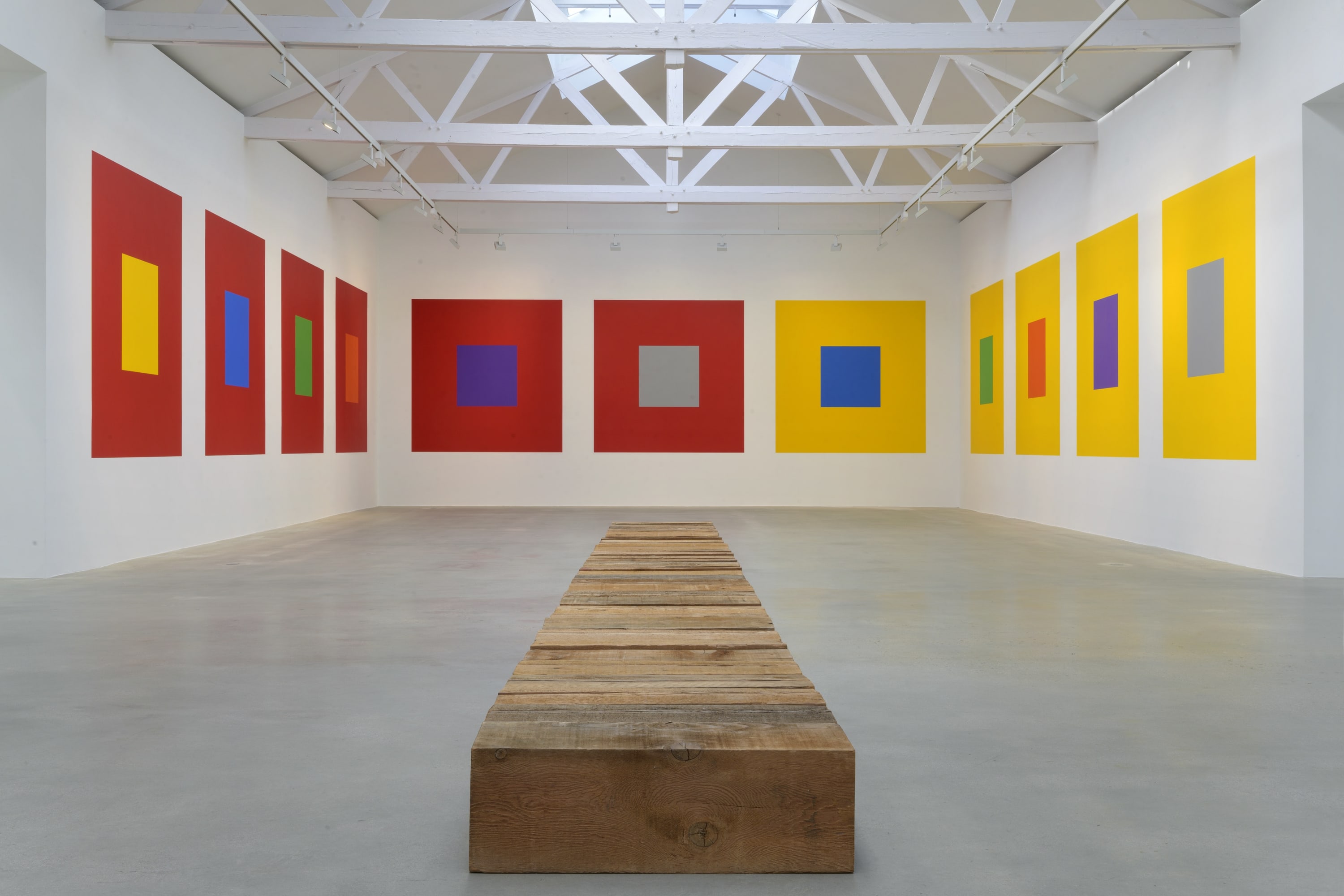The image depicts the interior of an art museum with an empty room that has a grayish-white concrete floor and white-painted walls. Each wall is adorned with painted square artworks showcasing a striking use of color. 

On the left wall, there are four large red squares, each containing a smaller square painted in yellow, blue, green, and red. The central wall displays three squares: the first is a large red square with a purple small square, the second is a large red square with a gray small square, and the third is a yellow square with a blue small square. The right wall features four yellow squares, each inscribed with smaller squares in green, red, purple, and gray.

A substantial wooden bench, resembling a slab or plank, extends down the center of the room's floor, indicating a place for visitors to sit and contemplate the artwork. The room's ceiling is sloped and fitted with white-painted metallic beams, further emphasizing the industrial and modern aesthetic of the space.